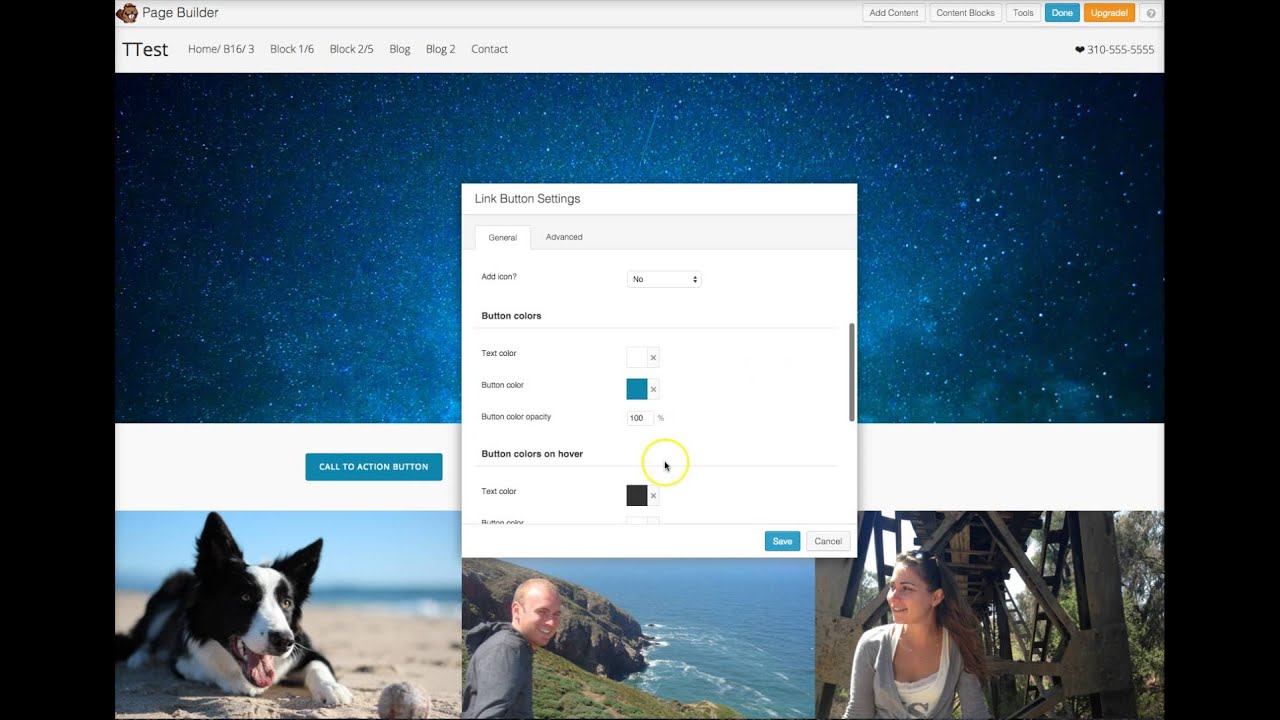This screenshot captures a detailed view of a web page, likely related to a content management or website building tool. 

At the top of the page, a small icon resembling either a beaver or a bird is paired with the text "Page Builder." This top ribbon includes several buttons labeled: "Add Content," "Content Blocks," "Tools," "Done," and "Upgrade." Adjacent to these buttons is a grayed-out question mark icon, presumably a help button. Just below this, another ribbon features the text "T TEST" in uppercase letters, followed by several navigational links: "Home /b16/3," "Block 1 /6," "Block 2 /5," "Blog," "Blog 2," and "Contact." On the far right side of this ribbon, a heart icon accompanies the phone number "310-555-5555."

The background of the webpage presents an evening sky, darkening from a bluish center to black around the edges, decorated with a starry night theme.

Centrally located on the screen is a pop-up box labeled "Link Button Settings." The currently selected tab is "General," with "Advanced" being the unselected option. Within the "General" tab, the first option is "Add Icon," set to "No." The next section, highlighted in bold, is "Button Colors." Here, "Text Color" is set to white, likely the default option, while "Button Color" is turquoise blue and set to 100% opacity. Another section labeled "Button Colors on Hover" appears below, but the content is partially obscured. A yellow circle surrounds the cursor pointer midway through the section divider. The visible setting shows "Text Color" set to black, and additional items below extend off the page as the menu is only halfway scrolled.

At the bottom of this pop-up box, two buttons are present: "Save," in the same turquoise blue as the button color, and "Cancel," which is grayed out.

Below this pop-up menu, three photographs are aligned horizontally. The first image features a black and white dog lying on a beach beside a baseball. The second picture shows a man standing on a cliff overlooking the ocean; he is smiling at the camera with light behind him. The third photo depicts a young girl wearing a gray top over a white t-shirt. She has brown hair with sunglasses perched on her head and appears to be standing in front of a metallic structure, resembling the base of a bridge.